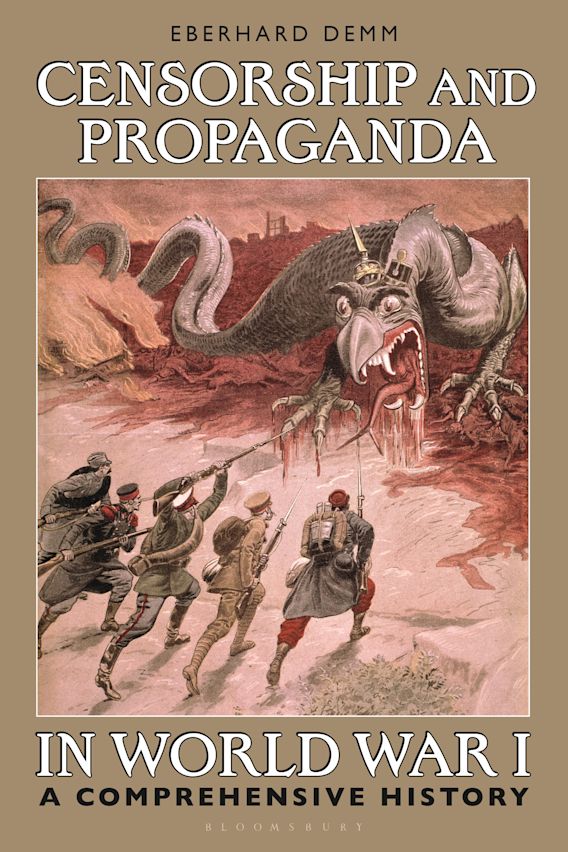The book cover for "Censorship and Propaganda in World War I: A Comprehensive History" by Eberhard Demme, published by Bloomsbury, features a dramatic and detailed illustration. Set against a tan-colored background, a dominating central image captures attention: a large, menacing dragon with its mouth wide open, displaying sharp, white fangs and a red tongue. Burgundy blood seeps from both its jaws and claws, staining the ground beneath. The dragon, colored in blood-like hues and adorned with a gold turreted helmet, exudes a sense of danger and ferocity. In the foreground, five soldiers, each in distinct World War I-era uniforms representative of different nations, charge courageously towards the dragon, their rifles with bayonets pointed menacingly. Their uniforms feature shades of grey with touches of red, and one soldier stands out in brown. The scene unfolds under a red sky, with a barren, bleak landscape devoid of life and positivity stretching out behind the dragon. The book's title and author are prominently displayed above this intense tableau, with the publisher's name, Bloomsbury, subtly printed in small white text at the bottom.